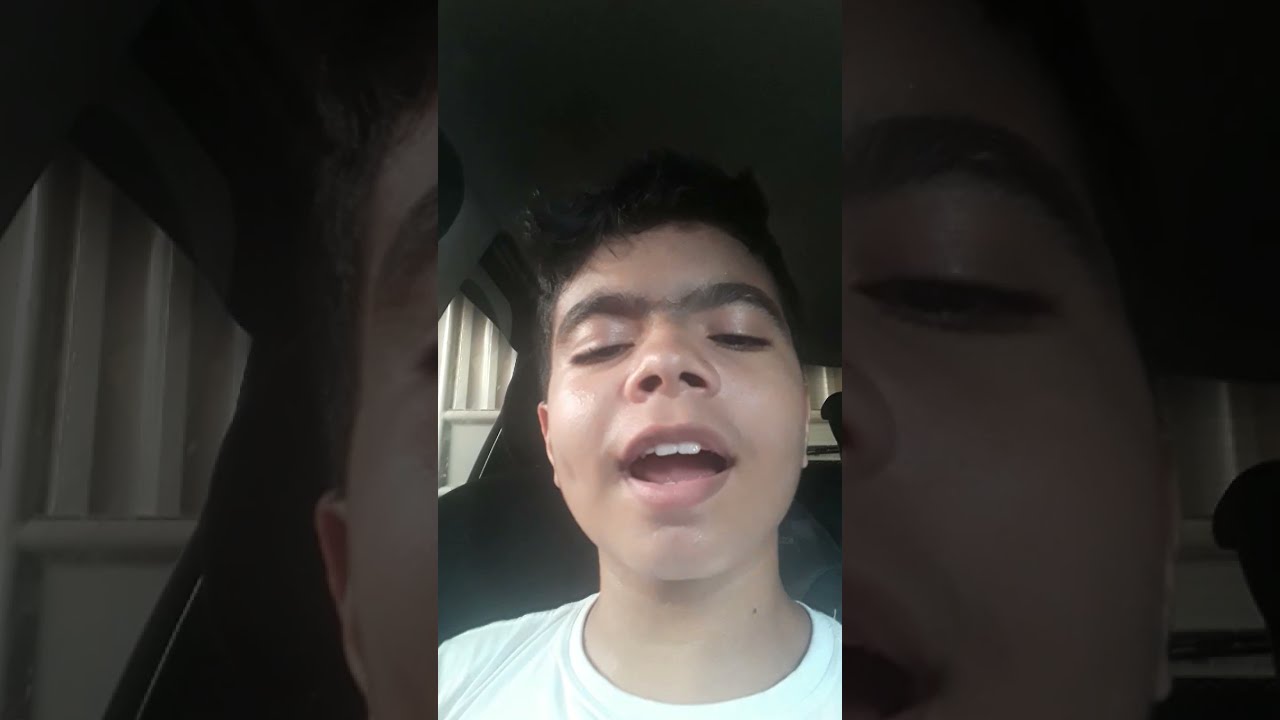In this vertical image, a young boy, likely of Mexican or Puerto Rican heritage, is taking a selfie or a thumbnail for a video. He appears to be around 14 or 15 years old, with short, black hair and notably thick, almost unibrow-like eyebrows. His eyes are half-open, and his mouth is open, revealing his two front teeth. The image seems to be a screenshot from a video, possibly captured on an iPhone and potentially posted on social media. He is wearing a white t-shirt and is seated in a vehicle's front seat. Behind him, the vehicle's interior features can be seen, including car windows and a ceiling that is black or gray. The scene outside the car shows thin, white pillars against a beige background, suggesting the vehicle is backed against a wall, perhaps near a warehouse or place of work. Additionally, his face is superimposed on both sides of the image.